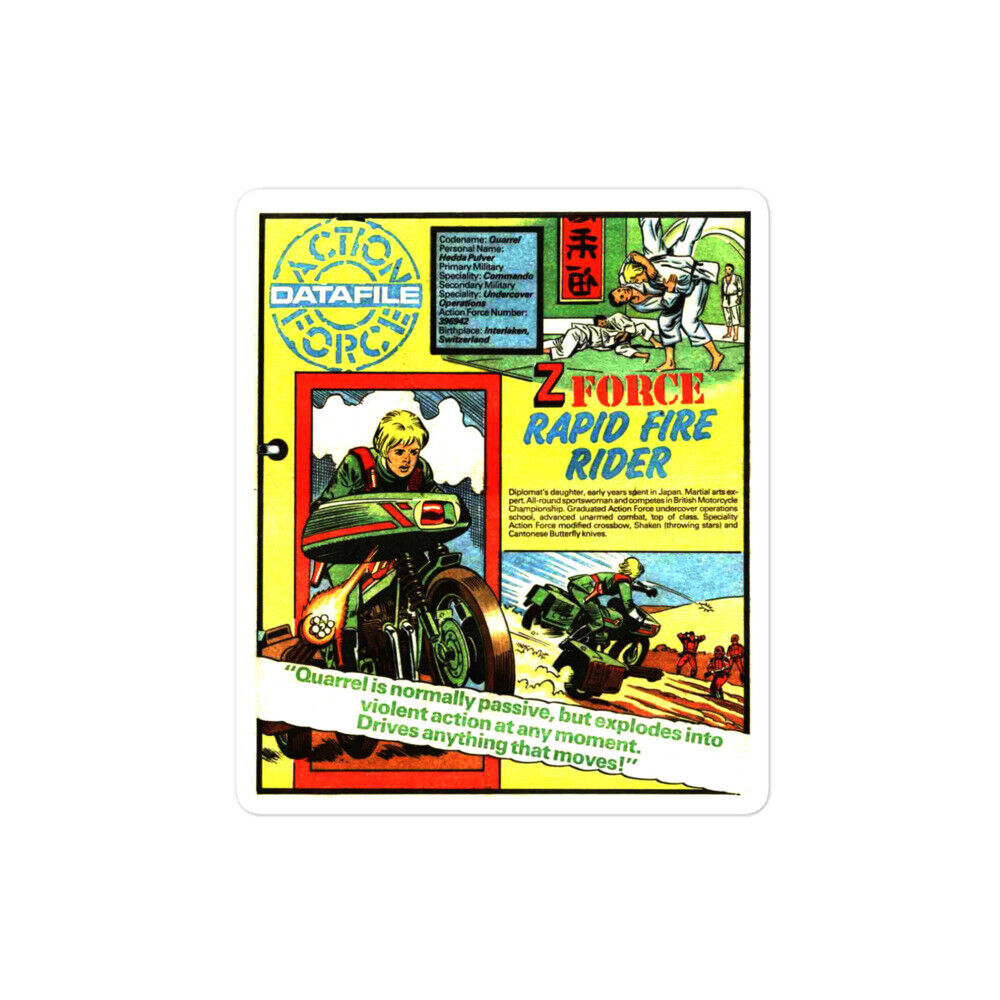The image is a portrait-oriented, color-printed comic book page featuring various vibrant illustrations and text. Dominating the background is a bold yellow hue. In the top left corner, there is a circular blue-stenciled logo, with "Action" across the top, "Force" around the bottom, and an aqua horizontal stripe across the middle with white text that reads "Data File." 

In the top right corner, a colorful comic panel depicts several people practicing judo or karate in a room, wearing white uniforms and engaging in dynamic martial arts moves. Adjacent to this, a red banner with Asian writing runs vertically beside this scene. Below this panel, the words "Z-Force" appear in red text, and beneath that, "Rapid Fire Rider" is boldly written in blue.

On the left side of the page, another panel illustrates a young man riding a green motorcycle. This same character reappears in a panel at the bottom right, now engaged in an intense action scene. He is mounted on the motorcycle, which is equipped with a machine gun, and is seen hurtling a grenade or similar explosive towards a group of enemies. Adding to the drama, a white strip with green text runs diagonally across the page, stating, "Quarrel is normally passive but explodes into violent action at any moment, drives anything that moves."

The overall style of the page is reminiscent of the classic comic book art from the 70s, characterized by its vivid color palette and dynamic action sequences.